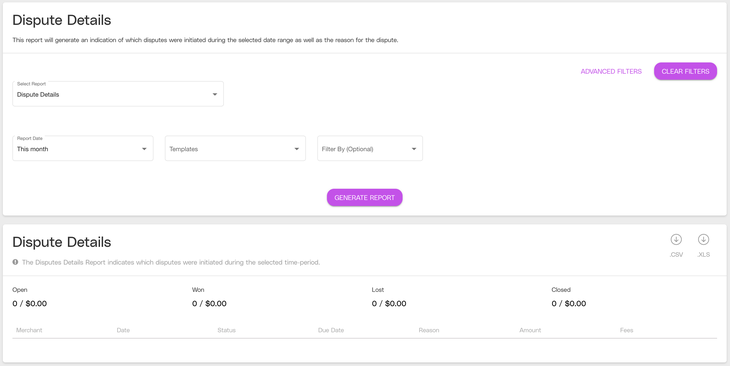This is a detailed screenshot of a website interface designed for disputing charges, such as credit card charges. The interface features two predominant sections, both encased in white boxes.

In the top section titled "Dispute Details," a description in small black text on a white background states, "This report will generate an indication of which disputes were initiated during the selected date range, as well as the reason for the dispute." Below this description, a gray horizontal line separates the text from the interactive elements below. To the right, purple text reads "Advanced Filters," followed by a pinkish-purple oval button with white text that says "Clear Filters." 

Adjacent to these elements, a dropdown labeled "Dispute Details" is present on the left. Three additional dropdown boxes are arranged vertically: "Report Date," which is set to "This Month," and two grayed-out options labeled "Templates" and "Filter by (Optional)." Centrally aligned beneath these dropdowns is another pinkish-purple button with white text marked "Generate Report."

The second section mirrors the first in structure and also begins with the title "Dispute Details" on the top left. A similar description follows: "This disputes detail report indicates which disputes were initiated during the selected time period." Below this description, metrics in black text are listed horizontally: "Open: 0 out of $0," "Won: 0 out of $0," "Lost: 0 out of $0," and "Closed: 0 out of $0." Underneath these metrics run a series of grayed-out column headers, categorically organized as "Merchant," "Date," "Status," "Due Date," "Reason," "Amount," and "Fees." However, all these fields are currently empty, indicating no data available for display.